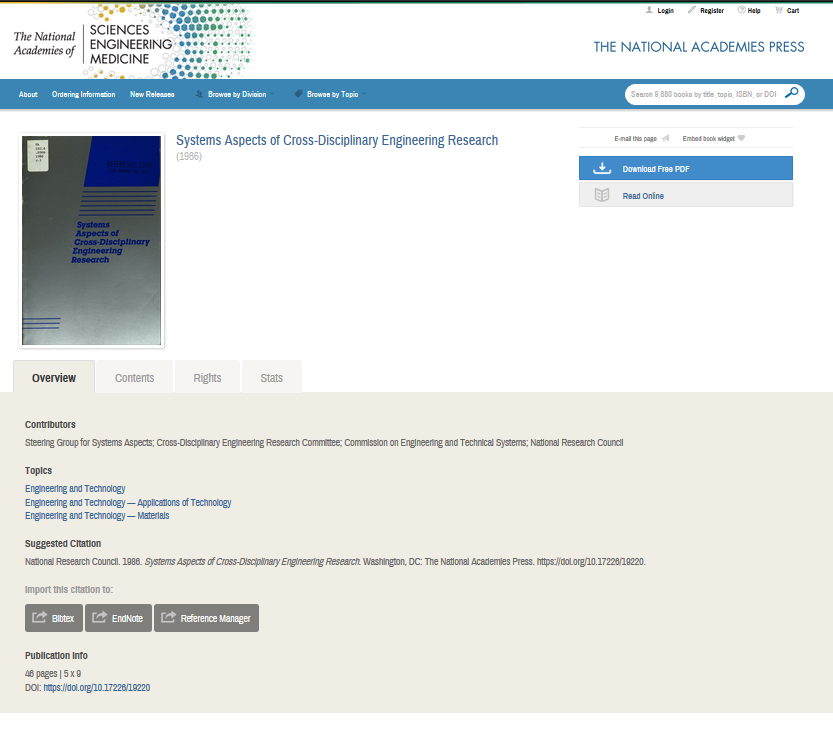The image depicts a web page from the National Academies of Sciences, Engineering, and Medicine. At the top, it features navigation options including "Log In," "Register," and "Help." The main section is titled "The National Academies Press," characterized by a large rectangular area. This section provides options to view "Boarding Information," "New Releases," and to "Browse by Division" or "Browse by Topic."

On the left side of the page, there's an option to search through "9,880 books by title, topic, ISBN," using Google. Below this, there's a section titled "Systems Aspects of Cross-Disciplinary Engineering Research," with a reference to "(19-6)." Additionally, options to "Email This Page," "Embed Book Widget," "Download Free PDF," and "Read Online" are visible.

The overview of the content includes sections on "Steering Group for Systems Aspects of Cross-Disciplinary Engineering Research," "Committee Commissions on Engineering and Technology Systems," and various aspects related to engineering and technology, such as materials and adaptation technology. The page also features a citation for the National Research Council and provides tools to import the citation to a reference manager. The content spans four to six pages and is formatted in a 5 by 9 layout.